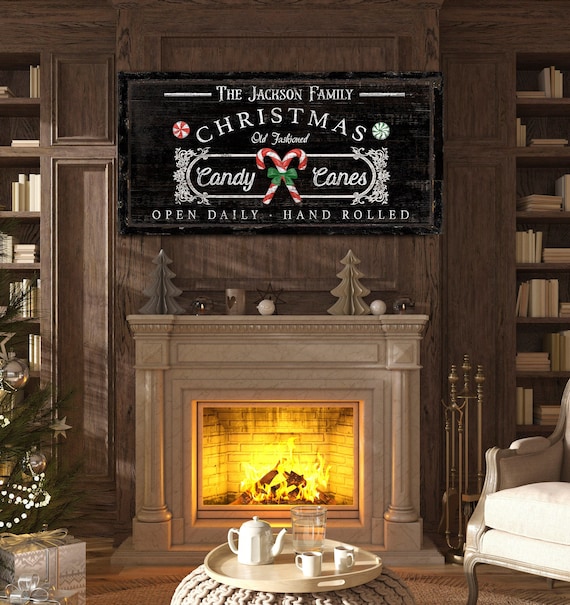The image depicts a cozy indoor residential living room centered around a lit fireplace with orange flames and burning wood. The fireplace, made of tan marble, is flanked by wooden bookshelves on both the left and right sides. Above the mantle, there is a large black sign that reads "The Jackson Family Christmas" with an oval design that contains the words "candy canes" and an image of crossed candy canes. Below, it reads "Open Daily, Hand Rolled." The mantle is decorated with two wooden Christmas tree ornaments, two candles, a cup adorned with a heart, and a few other decorative items. Directly below the fireplace, a white cushioned chair is positioned to the right, and to the left, there is a partially visible, decorated Christmas tree adorned with white pearls, stars, and lights, with a present underneath. In the foreground at the bottom center, a coffee table with a white tray holds a white teapot, two coffee mugs, and a water pitcher.